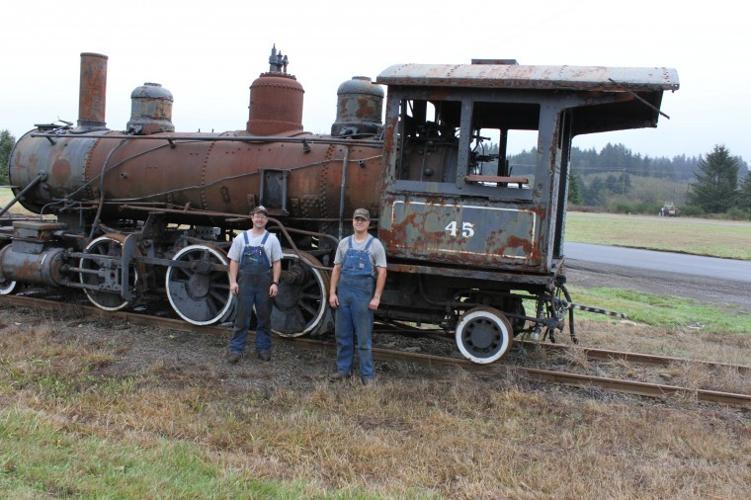The photograph showcases two stern-faced men standing in front of a very old, rusted steam locomotive numbered 45, which appears to be abandoned or at least out of use, evident from its heavy rust and wear. The locomotive is adorned with classic large driving wheels and a prominent chimney, typical of its vintage design. The men, dressed in denim overalls and hats, suggest they might be workers associated with this environment. The man on the left wears a light gray shirt, while the man on the right's shirt is a darker gray. The setting is an outdoor field with a mix of brown and green grass, surrounded by large trees and distant hills. Overcast, cloudy skies and the bright, natural daylight provide clear, well-lit visibility for the photo. The locomotive is situated on train tracks, facing left, with the men positioned right in front, enhancing the image's depth and context against the backdrop of the tree line and a nearby road.